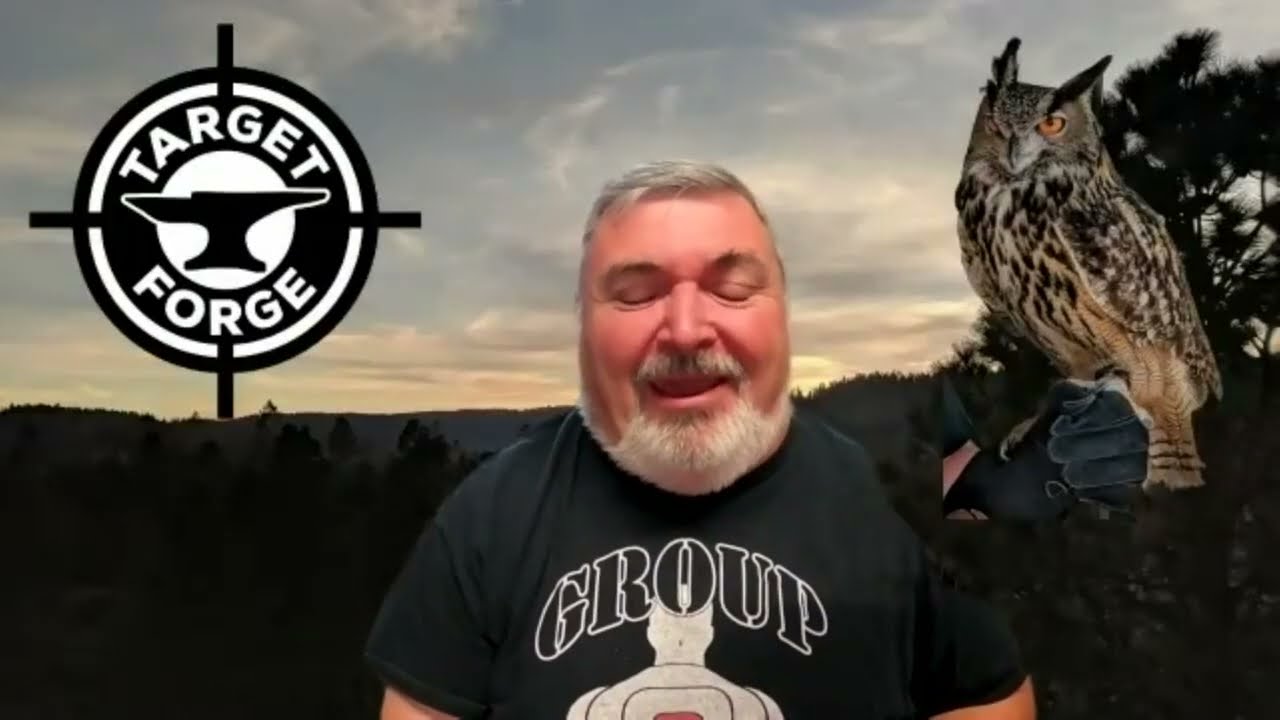In this detailed nature scene, an older man with thin gray hair parted to his left and a thick white beard takes center stage. His eyes are closed, and his mouth is open, as if he's speaking. He wears a black short-sleeved t-shirt emblazoned with the word "GROUP" in black font outlined in white. The shirt also features a partially visible graphic of a broad-shouldered figure with a target symbol on the shoulder, and the words "TARGET FORGE," along with an anvil emblem, are evident.

In his left hand, the man holds up a spotted owl with distinctive brown and white plumage, perched securely on a special glove. The owl's head is gray with striking yellow eyes and black-tipped ears. The backdrop behind the man has the appearance of a green screen, displaying a dense ridgeline of evergreen trees leading up to a sky that's grayish-blue, adorned with white, wispy clouds. This combination creates an evocative, serene forest setting that enriches the overall atmosphere of the image.